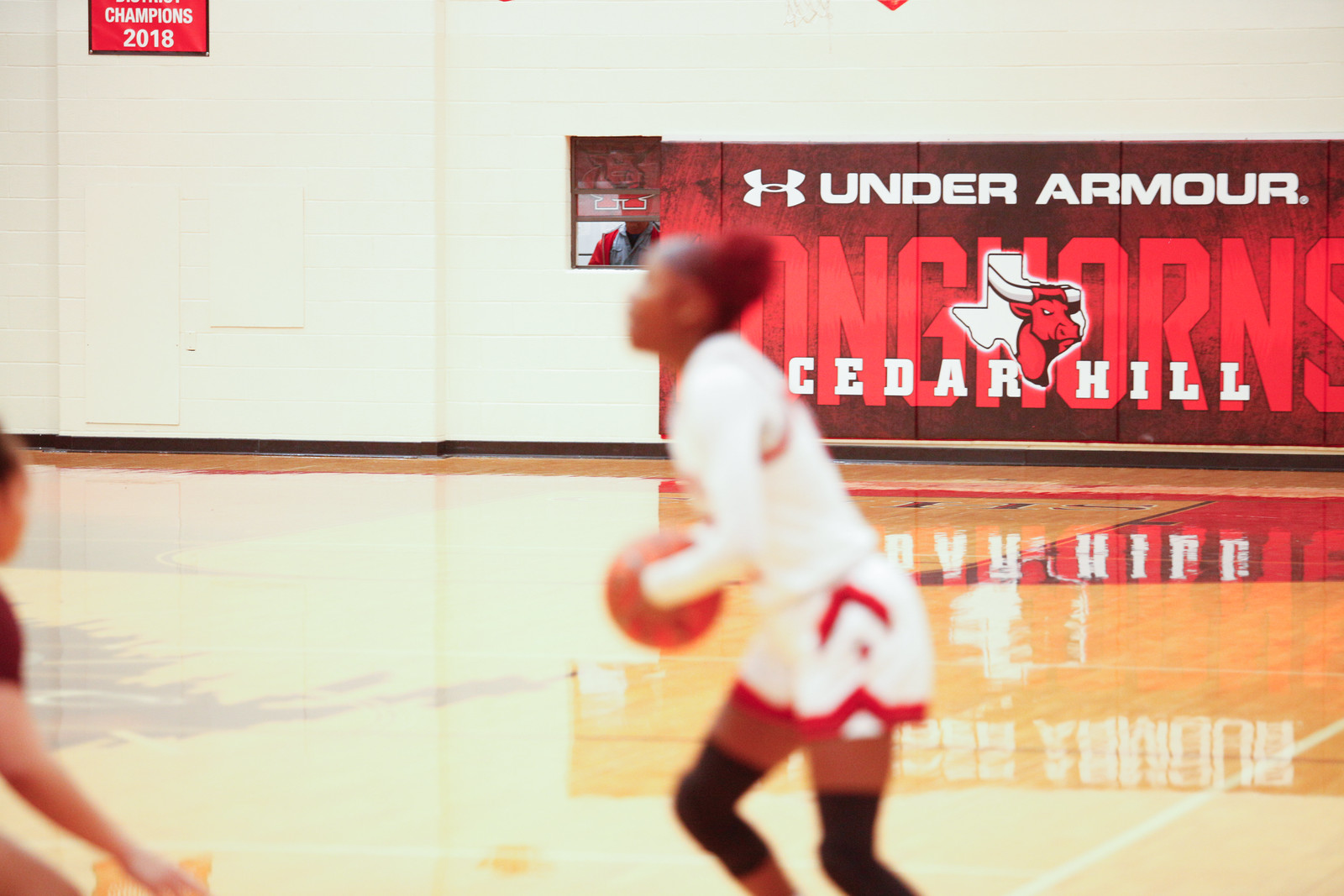This photograph captures a dynamic moment at a high school girls' basketball game in Cedar Hill, Texas, featuring the Cedar Hill Longhorns team. Central to the image is an African American girl in a white jersey with red accents, branded by Under Armour, poised to take a shot. She wears knee braces on both legs, underscoring the intensity and physical demands of the sport. Though slightly out of focus, her presence is dominant against the vividly detailed background.

The gymnasium walls are adorned with red and white impact mats, emblazoned with the Under Armour logo and the words "Longhorns Cedar Hill," accompanied by a Texas state emblem with a longhorn bull. The floor is polished to a high shine, reflecting the logo and contributing to the overall vibrant atmosphere. In the backcourt, a ticket booth is staffed by a gentleman, adding a touch of human activity and suggesting that this is a well-attended event. The image also indicates that the team achieved some level of championship status in 2018, although the specific title is not entirely clear. The photograph not only highlights the athletic prowess of the players but also the strong community and brand support behind them.